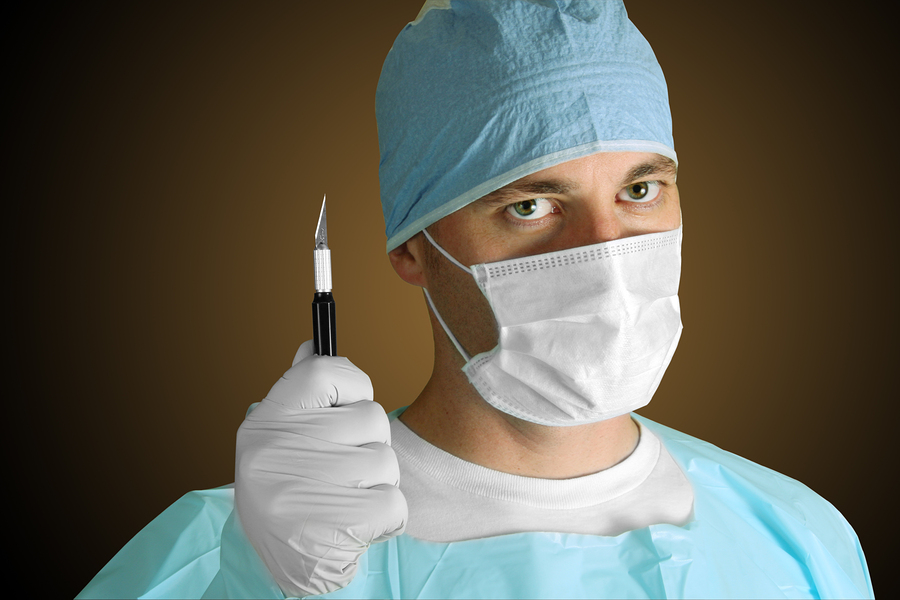The image captures a close-up of a surgeon from the shoulders upwards, set against a gradient brown background that darkens to black at the edges, drawing the viewer's focus to the center. The surgeon is dressed in full surgical attire including a light blue medical smock over a white crew-neck t-shirt, a blue scrub hat, and a white cloth mask with ear loops. His expression is intense as he looks directly at the camera. His right hand, clad in a white latex glove, is raised and gripping a scalpel with a black handle and a sharp, triangular-shaped silver blade. Bright lighting accentuates the surgeon, highlighting his green eyes and bushy eyebrows, and casting subtle shadows on his neck, making him the focal point of the image, possibly indicating a pre-surgery setting.